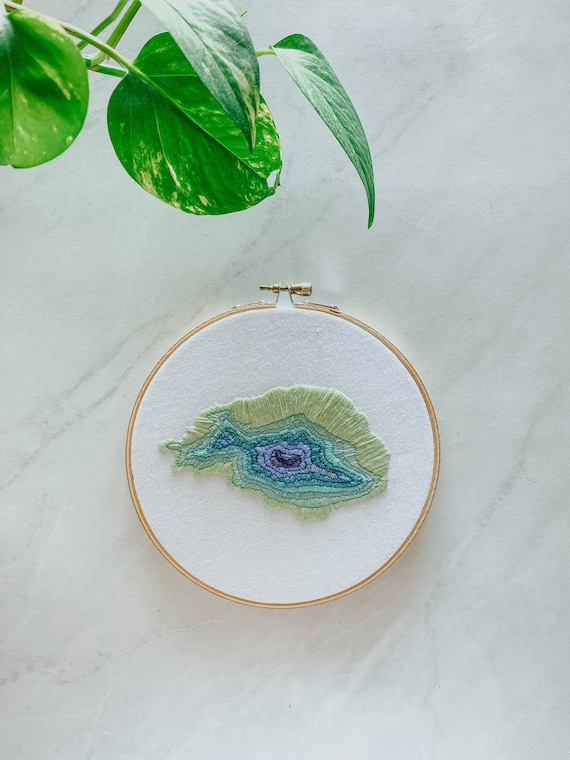The image features a close-up of an ornate, circular object framed by a gold rim, prominently displayed against a white background. Central to the object is an intricate mosaic design resembling a fish, radiating from the center in increasingly larger segments. The fish starts with a deep purple center and transitions outward through shades of lilac, blue, teal, and finally pale green tiles. This detailed mosaic fish is oriented towards the right side of the image.

Surrounding the fish are four bright, shiny green leaves with little green stems, suggesting the presence of an ivy plant. These leaves are positioned toward the top left corner, adding a natural frame to the scene.

The gold-rimmed object, possibly an earring or the cover of a makeup case, includes a gold screw-like fixture at the top, indicating it might also be a sewing hoop. The entire composition rests on a white surface with subtle gray streaks, resembling a marble countertop.